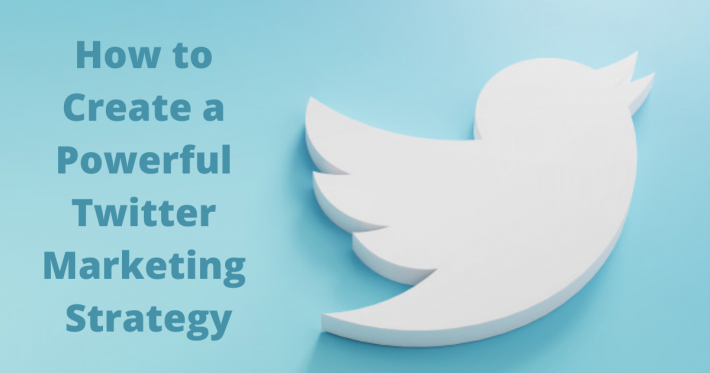In the image, there is a prominent Twitter logo featuring a white bird with wings extended and beak open, a departure from the usual blue color. The bird's shadowed elements add depth against the solid blue backdrop. Above the logo, bold blue text reads, "How to Create a Powerful Twitter Marketing Strategy," emphasizing the image's focus on strategic marketing. The entire visual composition is restricted to a blue and white color scheme, with blue used for both the background and the text, and white exclusively for the logo, creating a striking and cohesive look.